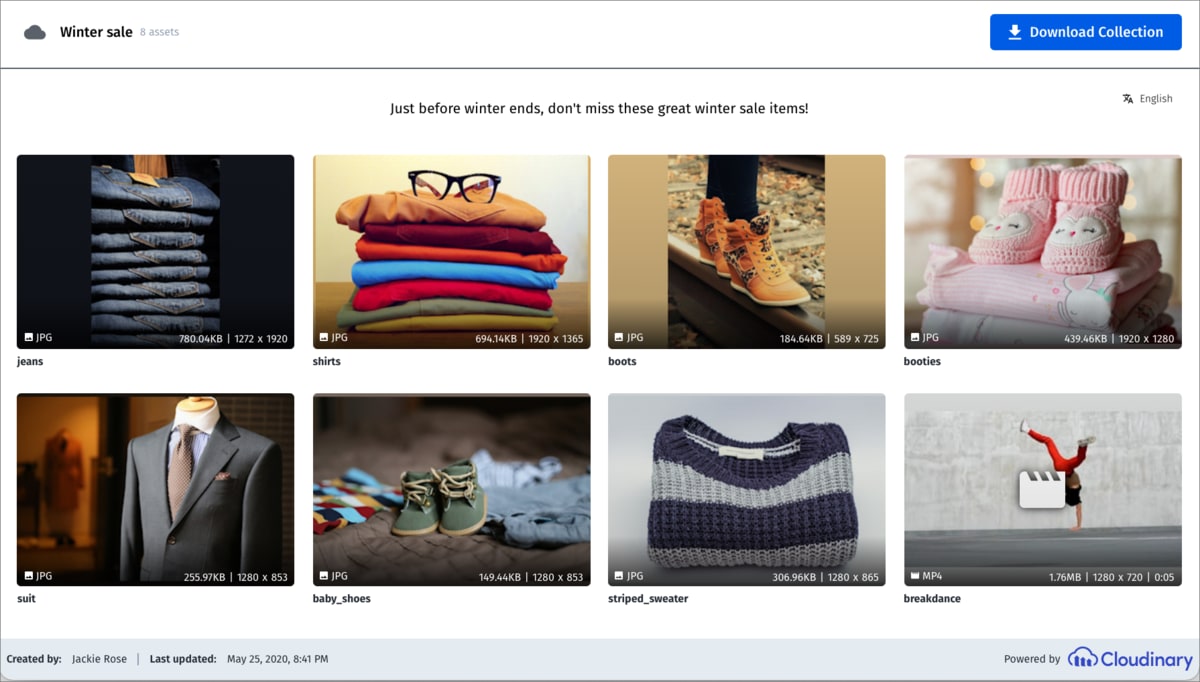An image depicting an e-commerce website's promotional page for a Winter Sale. The background is entirely white. In the upper left-hand corner, there is a black text heading that reads "Winter Sale." Positioned on the far right side of the page is a prominent blue button labeled "Download Collection."

Below the main heading, the page is divided into eight distinct tiles, each displaying a different product category. The first tile showcases a stack of jeans, reminiscent of a department store display, with the label "Jeans." To its right, the second tile is labeled "Shirts" and features an array of variously colored t-shirts stacked neatly, with an unexpected pair of eyeglasses placed on top.

Proceeding further to the right, the third tile presents a collection of boots, labeled "Boots." Adjacent to it, the fourth tile displays a set of booties, appropriately labeled "Booties."

The bottom row begins with the fifth tile displaying a formal suit, labeled "Suit." Next is the sixth tile featuring small baby shoes, labeled "Baby Shoes." The seventh tile depicts a striped sweater, easily identifiable though not explicitly labeled. The eighth and final tile is somewhat enigmatic and labeled "Breakdance," though its visual content is less clear.

At the bottom of the page, a banner includes the texts "Created By" and "Last Updated," with the far right corner of the page indicating "Cloudinary, Prepared By Cloudinary."

Overall, the page is characterized by its clean, minimalist design, with a focus on the eight product categories against a stark white background.